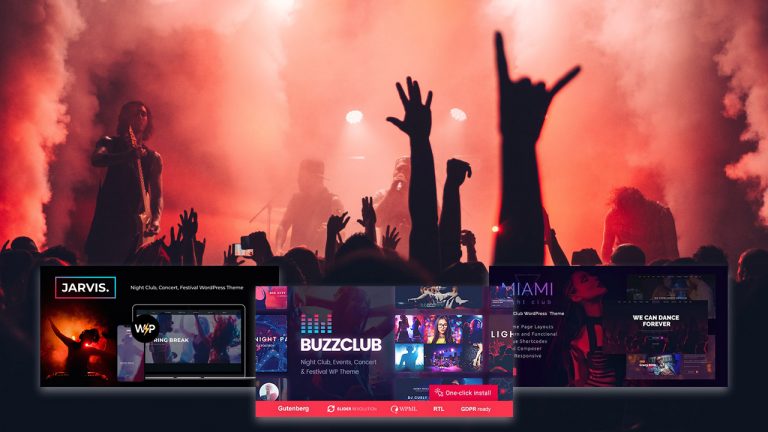The image captures the dynamic atmosphere of a live concert. On stage, several singers and performers are energetically engaging the audience. The air is filled with a dramatic plume of steam, creating an immersive and vibrant experience. Overhead, brilliant beams of light descend from the ceiling, illuminating the performers and creating focal points of intense brightness.

In the forefront, prominent signage displays the name "Jarvis" in bold letters. Additional advertisements flank this central text, including tags such as "Jarvis," "Buzz Club," and "Miami," suggesting a promotional event for these brands or locations. 

A red line at the bottom of the image indicates interactive categories, presumably part of a digital interface, offering clickable options.

In the crowd below, the silhouettes of audience members are animated in the darkness, with many hands raised high. Some hands are wide open, fingers splayed, while others form enthusiastic gestures with only the index and pinky fingers extended.

The lower portion of the image is a sea of black, dotted with the blurred shapes of concert-goers, adding depth and a sense of vastness to the scene. The overall effect is a captivating snapshot of the electrifying energy and communal joy of a live musical performance.